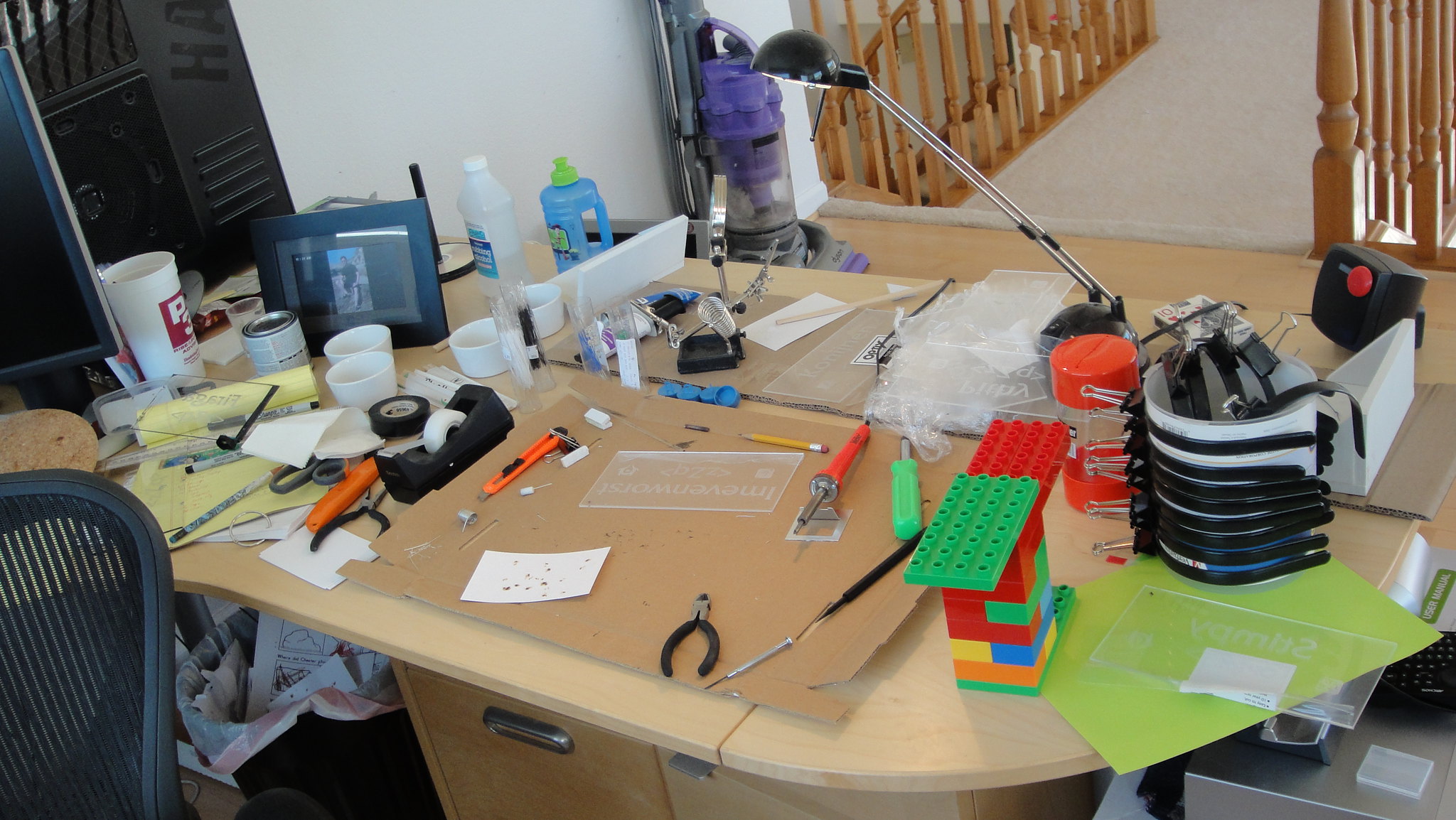The image is a color photo taken from above, showcasing a well-used desk. The desk is an unusual, deep shape, made from light-colored birch-wood or a similar material. Its rounded edges form a half-circle, ensuring safety from sharp corners. 

On the right side of the desk stands a colorful tower of Legos, featuring vibrant red, green, blue, yellow, and orange blocks. Beside it, a black-topped gooseneck lamp, likely an old halogen model but hopefully LED, arches over the workspace. 

The left side of the desk holds an orange slide-open X-Acto knife with snap-off blades, along with a cluster of cups and a small can with a lid, possibly for PVC glue. This section also includes an old-fashioned black Scotch tape dispenser, various tools including a pair of scissors, and a legal pad. 

Towards the right front, small snip-type pliers lie adjacent to a screwdriver with a lime-green handle and what appears to be a soldering iron on a stand. A sheet of material, potentially plexiglass or translucent paper, occupies part of the desk, alongside a number two pencil.

Amidst the clutter, a blue and green plastic bottle, possibly containing isopropyl alcohol, adds a touch of color. On the floor to the far side of the desk, a purple and gray upright vacuum cleaner with a HEPA filter stands, indicative of a tidy space beyond the desk’s surface.

In the background, a set of stairs descends, with a stair rail and newel posts visible against the wall-to-wall carpet. This suggests the desk is positioned in a small office area located on the top landing.